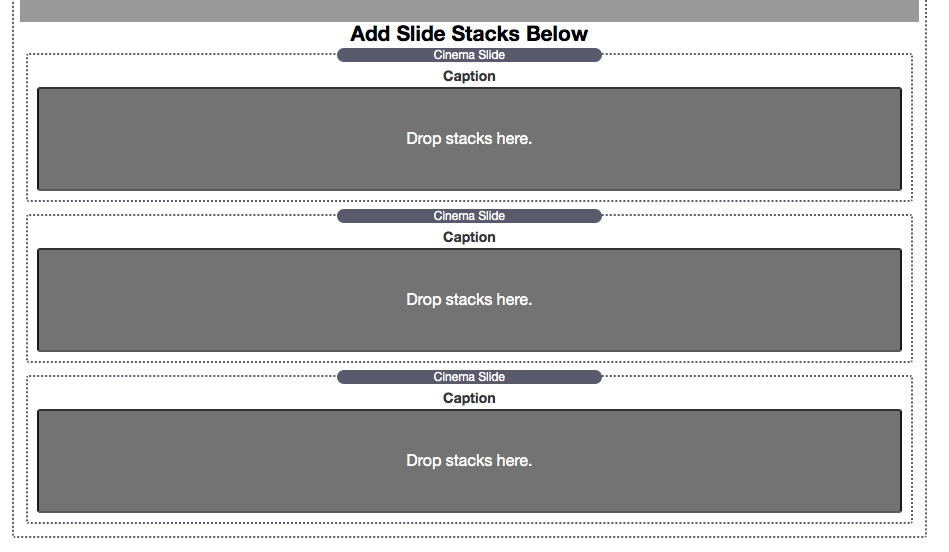The image features a series of organized sections and buttons framed by dotted lines and solid-colored boxes. At the top, there is a thin, dark gray box. Just beneath this box, bold, black text reads "Add Slide Stacks." Below this is a rectangular area outlined by a dotted line, within which there is a prominently colored, dark purplish section labeled "Cinema Slide." Under the "Cinema Slide" label, the word "Caption" is displayed. 

Following this, there's a box containing the instruction "Drop Stacks Here," also demarcated by a dotted line. Another similar structure follows: it starts with a label "Cinema Slide" with "Caption" beneath it, then transitions into a dark gray, rectangular box that reads "Drop Stacks Here" in white letters.

Continuing down the image, another rectangular section is outlined by a dotted line. At the top of this section, there is a dark purple button labeled "Cinema Slide," followed by the word "Caption" just below it. In the middle of this final section, a dark purple rectangle with white text instructs to "Drop Stacks Here," ending with a final line beneath it.